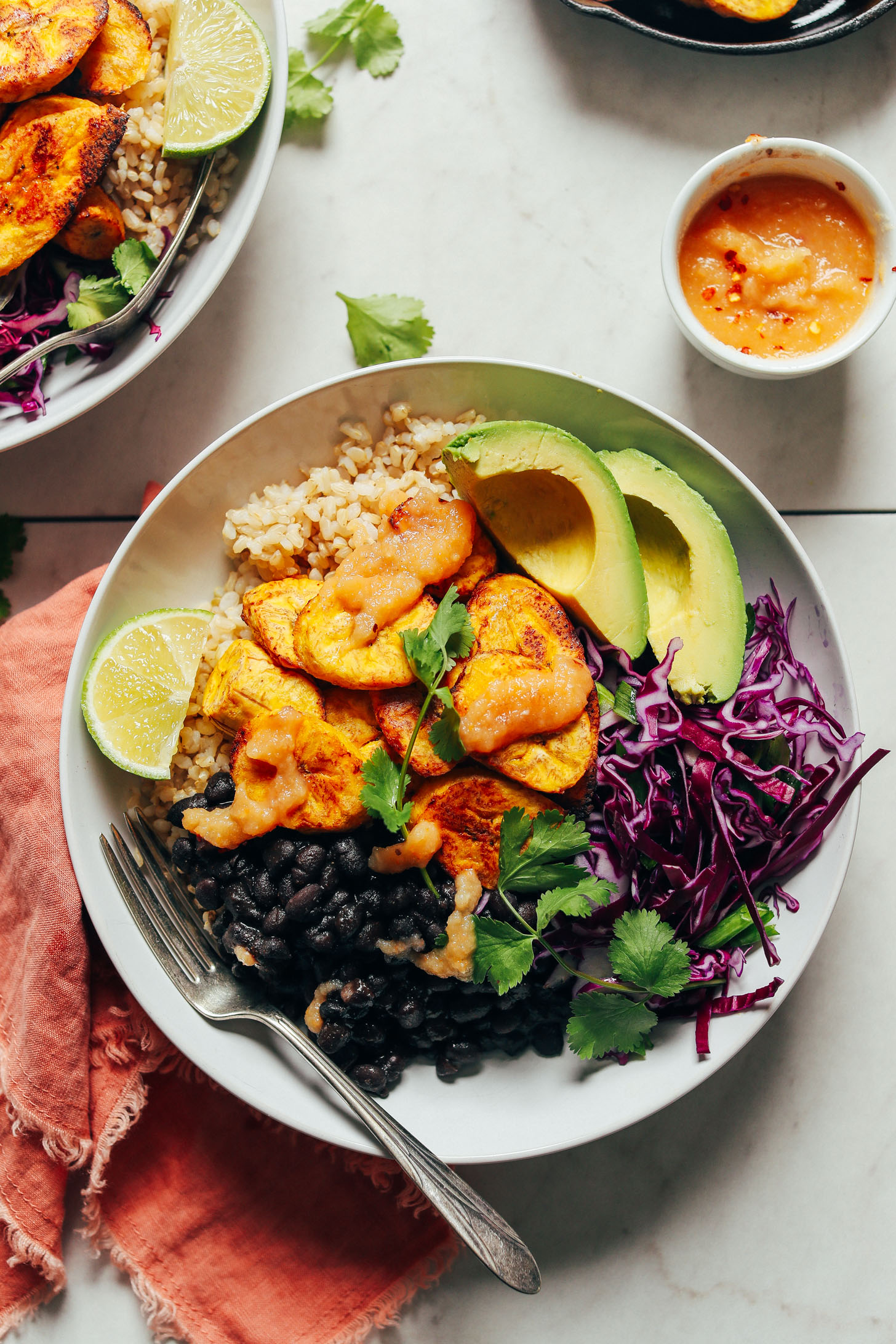The image depicts a vertically aligned, rectangular photograph, primarily showcasing a large white plate filled with a variety of foods, placed on a white marbled surface with a faint groove, indicating it could be either a countertop or floor tiles. Central to the composition is the white plate holding an array of delicious foods: light brown rice at the top, sliced avocados to the right, crusted shrimp in the middle, and shredded radishes alongside black beans at the bottom. Additional items include parsley leaves and a sliced lemon on the left. A silver fork is partly tucked under the black beans on the lower edge of the plate. Just beneath the main plate lies a crumpled, brownish-red dish towel with fringe. 

In the upper right corner, there’s a small, white condiment dish, possibly containing a tan-colored sauce with specks, and a partial view of another similar white plate in the top left corner. The main plate also seems to host purple onions and cilantro scattered throughout. A cast iron pan appears faintly in the distance, adding to the culinary context. This detailed, bird's-eye view arrangement portrays a harmonious and well-composed meal setting on a polished, white-and-gray, tiled surface.